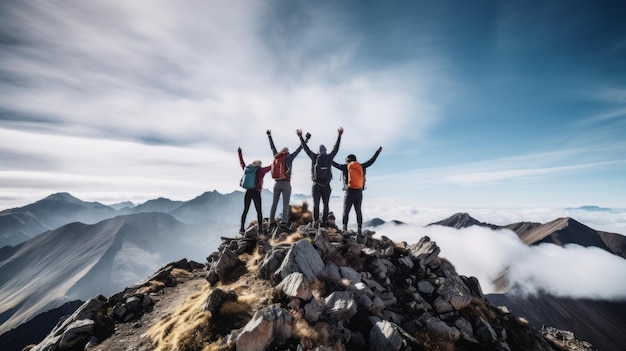In this captivating photograph, four adventurers stand triumphantly at the rocky summit of a high mountain, their arms raised in jubilant celebration of their achievement. The photo, taken from behind, shows them standing in a row on the rugged peak with backpacks of various colors - a blue, a magenta, a darker blue, and an orange. Dressed in pants and long sleeves, their figures are silhouetted against a panoramic backdrop of distant mountain ranges and patchy clouds that lie beneath them. Above, the sky is a brilliant blue streaked with wispy white clouds, encapsulating the essence of their lofty triumph.